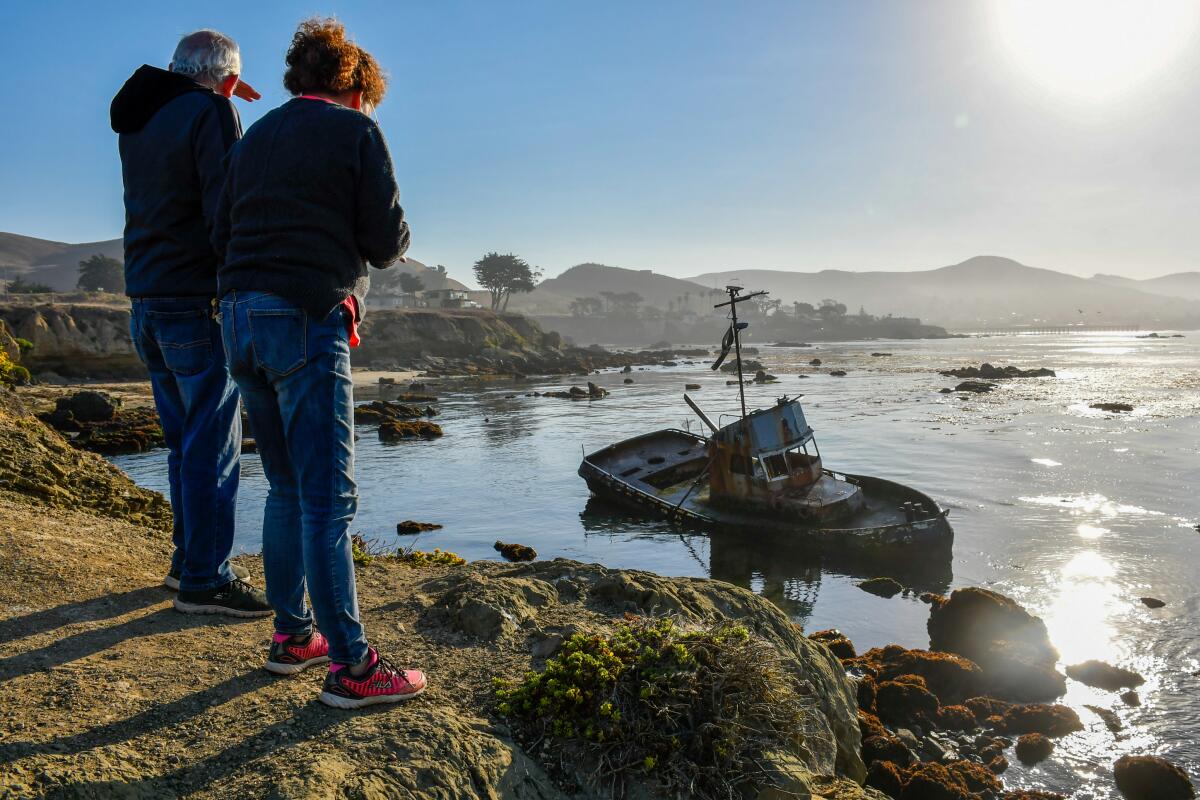This photograph captures a man and a woman standing on a dirt and gravel outcropping overlooking a picturesque bay. The woman, with red hair, is dressed in orange-red sneakers, blue jeans, and a black sweatshirt. Beside her on the left stands an older man with gray hair, wearing blue jeans and a black hooded jacket, shading his eyes with his hand against the bright sunlight. Below them, a dilapidated, half-sunken fishing boat rests in the dark, rock-studded waters. The shoreline curves into a mini peninsula, edged with sand and dotted with rugged, brown rocks. In the background, a serene landscape of hills and trees unfolds under the clear blue sky, with the sun shining brightly from the upper right.